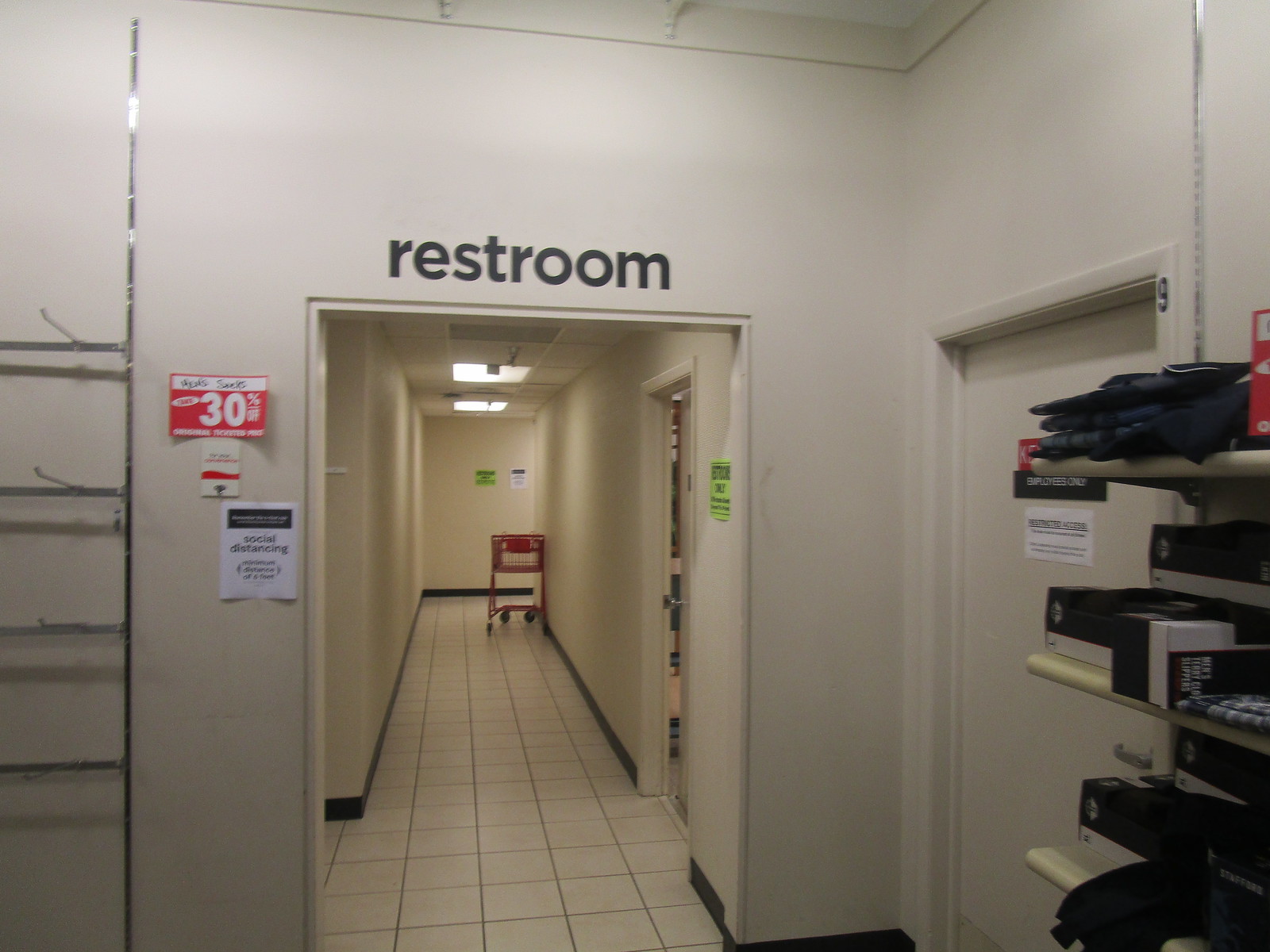This is a photograph of a hallway inside a store, leading towards a restroom area. The walls are off-white, and the floor is covered with square white tiles with black grout. Above a rectangular doorway, there is a sign that reads "restroom" in black letters. To the right, there are three beige-colored shelves mounted on the wall, displaying folded clothing items, including denim and black fabric pants, and several blue and white boxes. Just inside the hallway, a red shopping cart is parked against the right wall. To the left of the doorway, a silver ladder-like structure is leaned against the wall. Additionally, on the right, there is a door with a white sign on it, partially obscured by a silver metal bar extending behind the shelves.